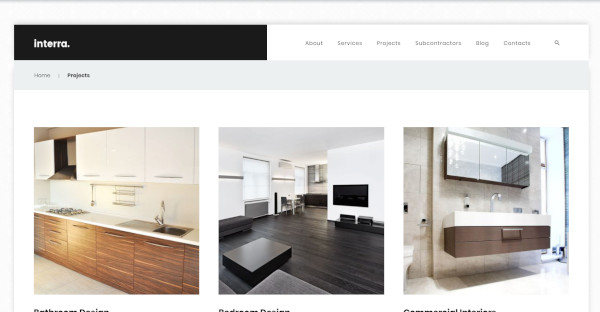This screenshot captures the homepage of the Interra website, albeit in a highly reduced size that makes the text somewhat difficult to read. The top navigation bar on the left features a black background with white text that spells out "Interra," occupying about a third of the width. To the right, the navigation menu stands out against a white background, listing the options: About, Services, Projects, Subcontractors, Blog, Contacts, followed by a magnifying glass icon for the Search function.

Directly below, a gray horizontal bar spans the entire width, presenting a set of breadcrumbs for navigation. It starts with "Home" on the left, followed by "Projects," indicating the current page.

The content beneath the navigation elements displays images of three highlighted projects. The first image on the left showcases a photograph of a sleek, modern kitchen. The design features white upper cabinets contrasted with wood lower cabinets. The middle image reveals a family room characterized by dark gray flooring, starkly modern square furniture, a large TV mounted on the wall, and several windows in the background providing natural light. Finally, the third image on the right captures a contemporary bathroom scene, featuring a wide floating vanity with a tall faucet, accompanied by several mirrors mounted above. The overall aesthetic emphasizes clean, modern design in each of these project images.